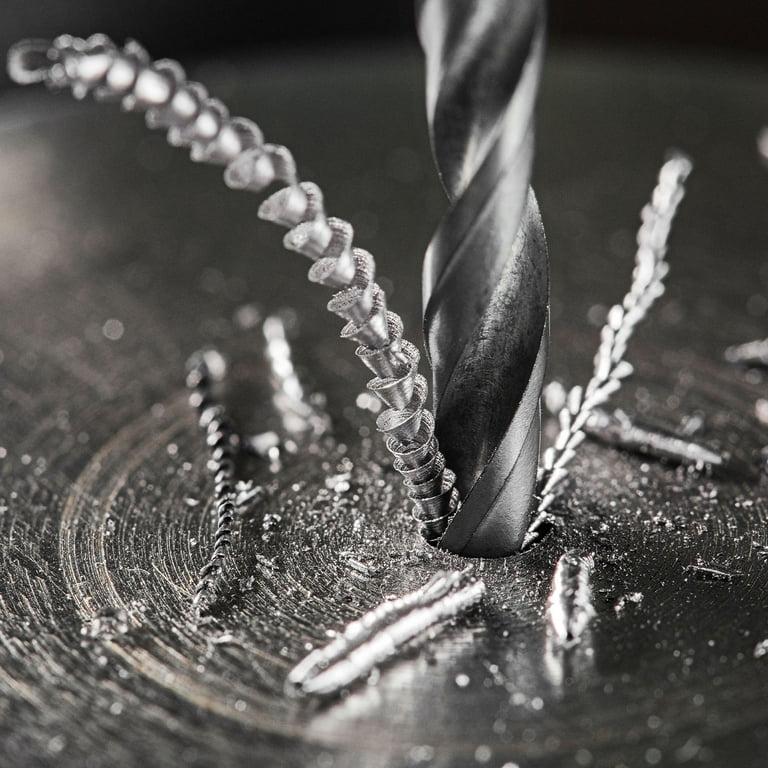This black-and-white close-up photograph captures the intense moment a drill bit penetrates a wooden surface. The grayish-black drill bit, with its detailed spirals running along its length, drives forcefully into the wood, causing a mesmerizing array of spiraled wood shavings to erupt from the newly-formed hole. These shavings, mixed with smaller wood chips, scatter across the wooden surface, creating a textured scene of displacement and activity. The drill's motion and pressure create a distinctive circular indentation in the wood, emphasizing the dynamic interaction between tool and material. The fine detail in the metal-like sheen of the wood shavings adds a contrasting visual texture to the organic grains of the wood, captured meticulously in this strikingly detailed photograph.